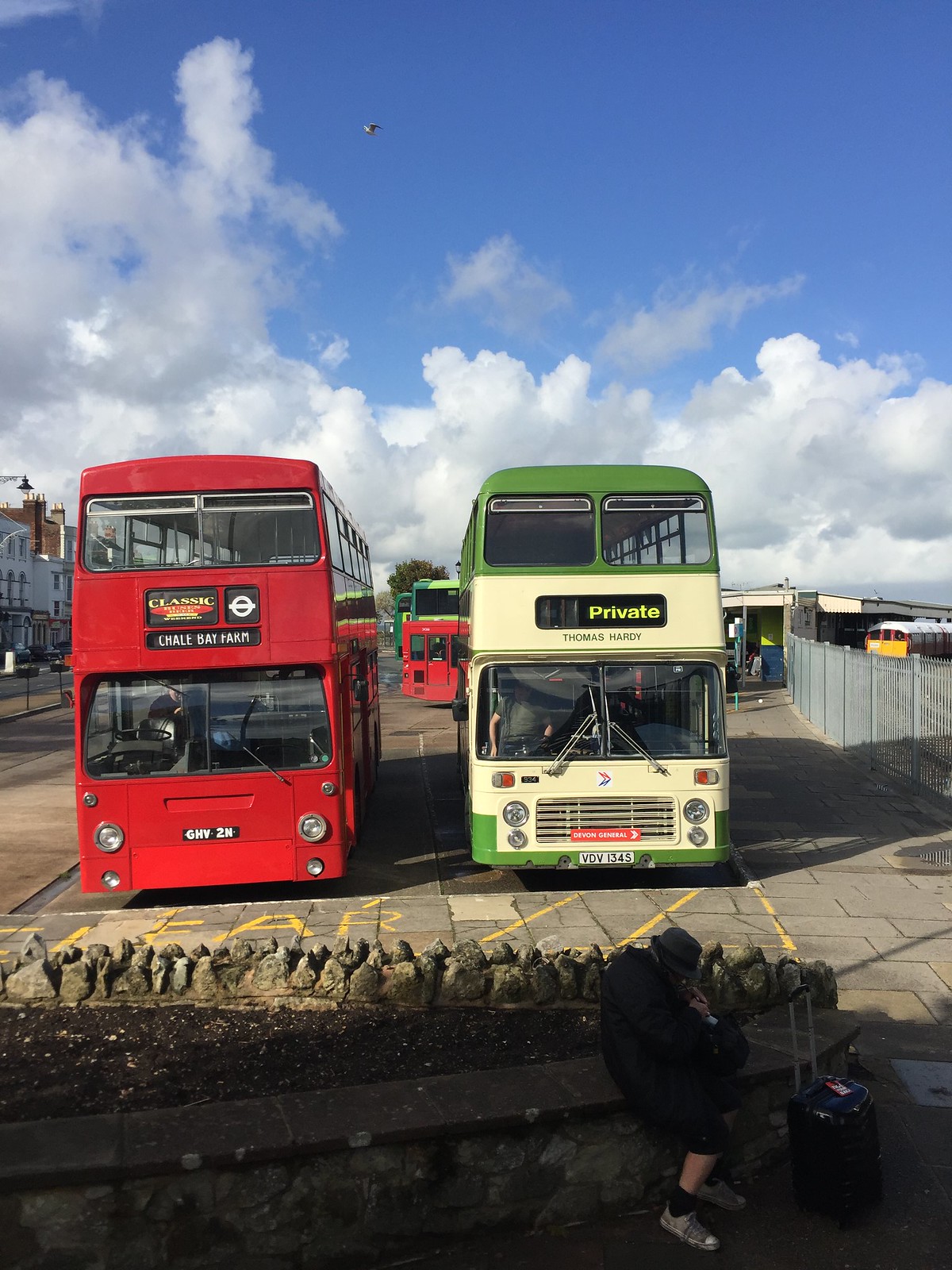The photograph depicts a vibrant outdoor bus stop on a sunny day with a deep blue sky and fluffy clouds overhead. Dominating the scene are two parked double-decker buses, one painted a solid red and the other green with a tan front. The red bus on the left displays the branding "Classic" and "Chale Bay Farm" in white text on a black background, with a black license plate reading GHV 2N. The green bus on the right is marked "Private" and "Thomas Hardy," along with a license plate VDV 1345. The red bus appears to be slightly taller, and the driver's seat of the green bus is occupied by a person wearing a short-sleeved shirt.

In front of the buses, a man sits on a low stone wall by the sidewalk, dressed in a hat, a dark tracksuit, and white tennis shoes. His face is obscured, and beside him is a roller luggage. Additional buses can be seen parked behind the main two, with buildings and fences receding into the background, hinting at a bustling town area. To the right, an iron post fence runs alongside railroad tracks, adding depth to the scene where a red and gold train is visible in the distance.